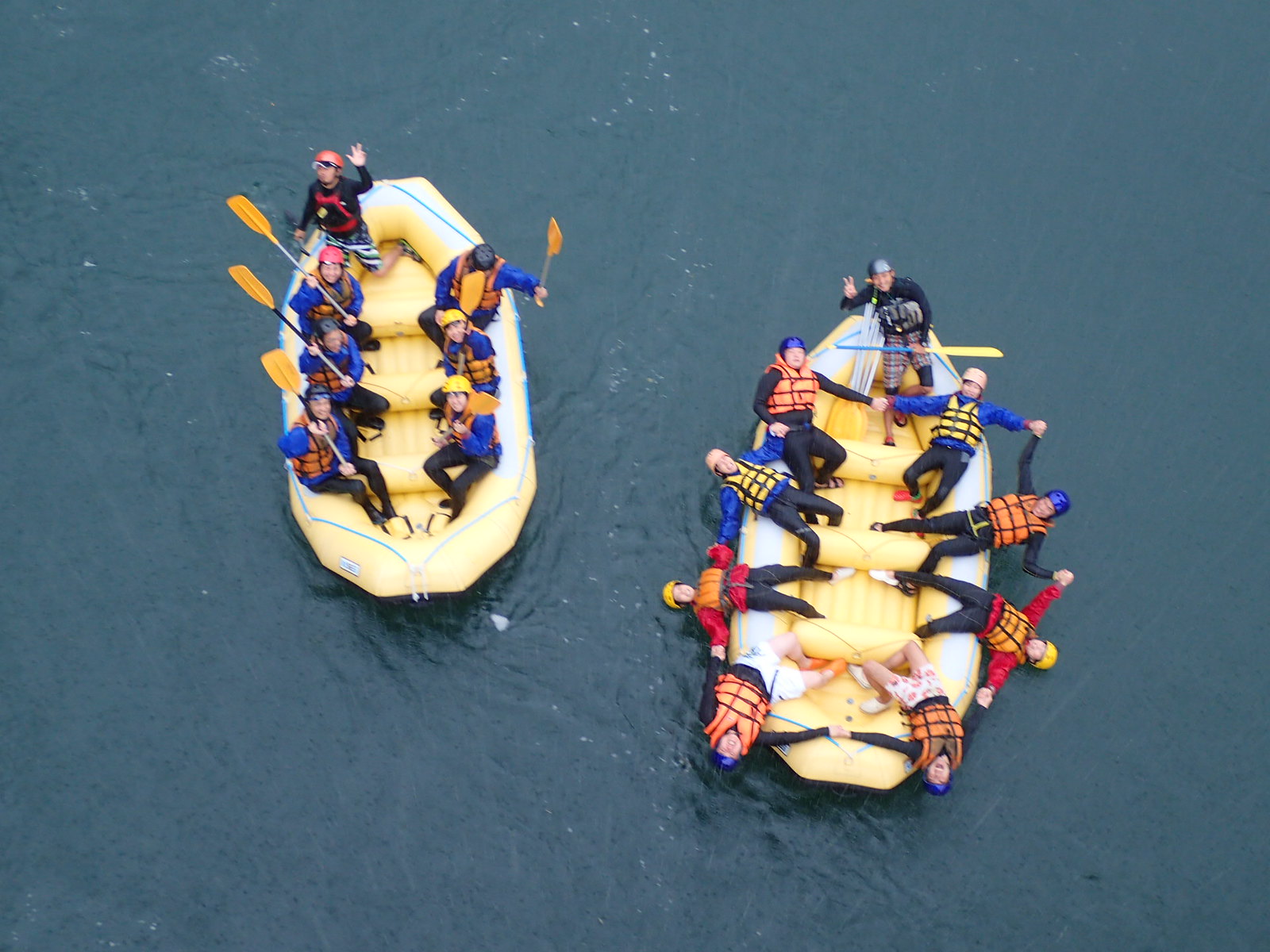In this digital photograph taken outdoors, the focus is on a dark, fairly still, blue body of water. Centrally placed in the image are two inflatable white dinghy boats. The boat on the left contains seven people, dressed predominantly in dark blue coats and black pants, with varying helmet colors: pink, black, yellow, and blue helmets. The person at the front left wears a black long-sleeve shirt and American-style swim trunks. 

The boat on the right also carries several people, dressed in a mix of blue, black, red, and orange jackets with matching helmets, along with black pants. Some individuals are leaning over the boat and holding hands. In this boat, there is a person standing at the back, dressed in red, who appears to be engaging with the camera and holding up a peace sign. Overall, the scene captures a diverse group of people partaking in an organized water activity on a somber-looking day, possibly under cloudy skies.